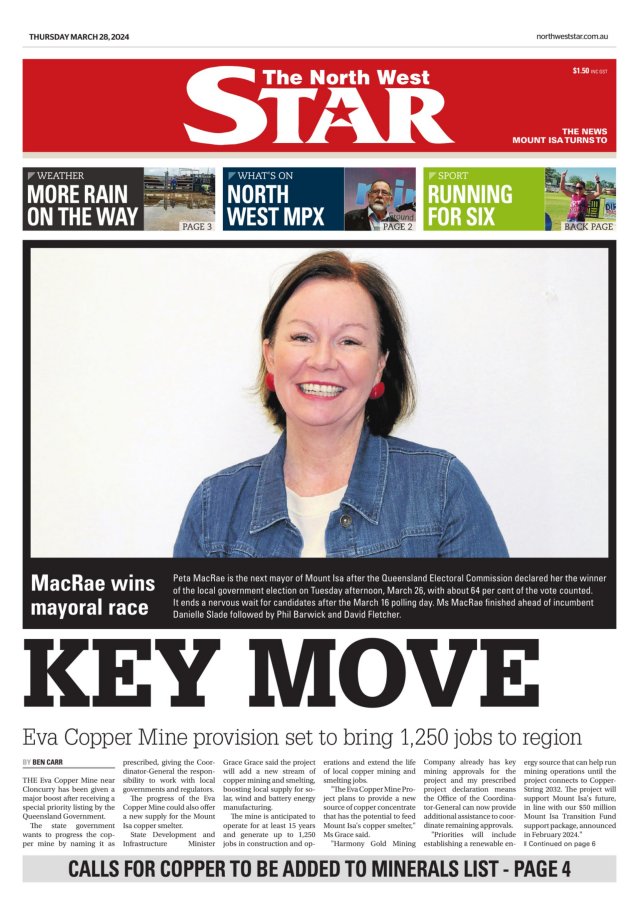The image depicts a cover of the "Northwest Star" magazine, identifiable by its title in large white letters with a star replacing the center of the letter "A." This particular edition appears to have been published on Thursday, March 28, 2024. Below the title, the cover features three primary headlines, each accompanied by corresponding images. 

The foremost headline on the left reads "More Rain on the Way," hinting at upcoming weather conditions. Adjacent to it, the middle headline states "Northwest MPX," followed by "Running for Six" to the far right. 

Dominating the cover is a prominent photograph of a smiling woman whose gaze meets the camera. This image is captioned in the lower left corner with "McCray wins mayoral race," indicating that she is the newly elected mayor. 

Beneath this central image, the phrase "Key Move" is displayed in bold, black letters, leading into an article titled "EVA Copper Mine Provision Set to Bring 1,250 Jobs to Region." Although there is additional text below this, it is illegible due to the small font size. 

At the very bottom of the cover, a brief note in black letters directs readers to "Page 4" for more information on the call to add copper to the mineral list.